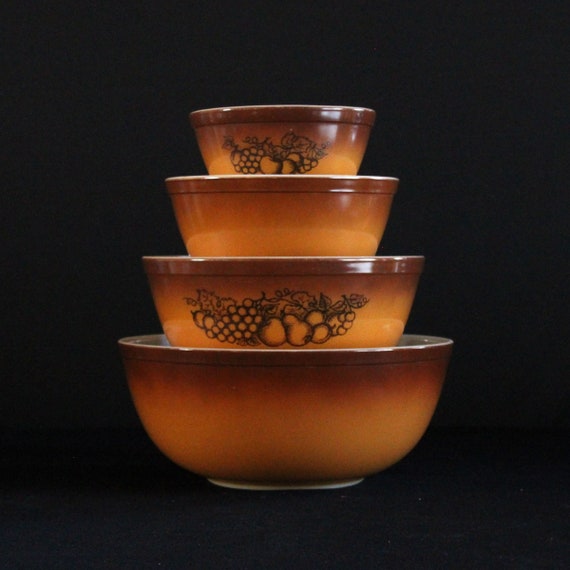The image showcases four nested bowls set against a pitch-black background. The bowls, arranged from largest at the bottom to smallest at the top, appear to be part of the same pottery collection and feature an earthy gradient that transitions from a rusty orange near the base to a darker brown at the rim. Each rim is delineated in white, contrasting with the white interior of the bowls. Notably, the largest and the smallest bowls display a simple yet detailed black outline drawing of a fruit arrangement, including grapes and pears, reminiscent of a cornucopia without the horn, an imagery often associated with harvests and Thanksgiving. The intermediate bowls, which are plain, allow us to observe the consistent coloration and subtle texture that might evoke a wooden appearance, though they are likely crafted from pottery. The bowls are not fully nested but rather stacked in such a way that much of each bowl remains visible, offering a clear view of their design and decoration.